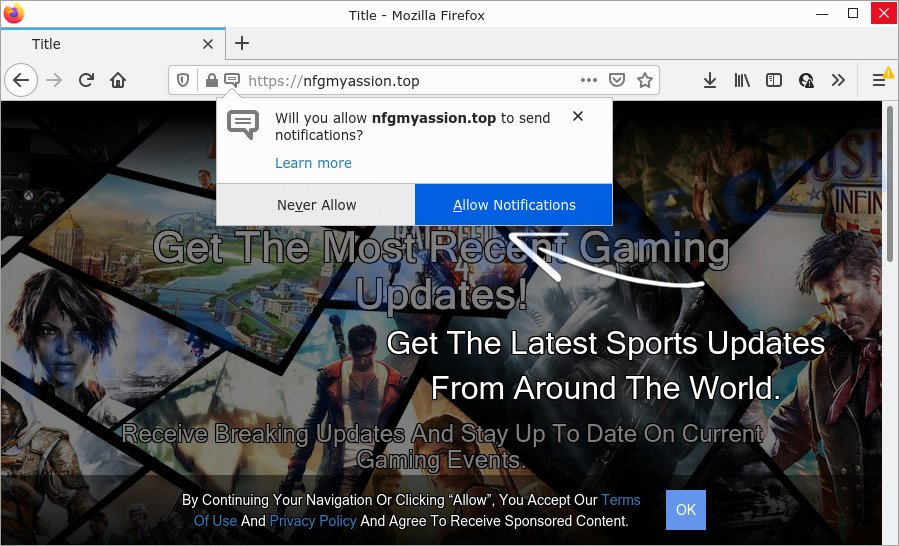Caption:

A detailed screenshot of a Mozilla Firefox browser window displaying a website with URL nfgmyassion.tlp. The top-left corner features the Mozilla Firefox logo, while the top-right corner contains the minimize, maximize, and close buttons. A single tab labeled "title" is open and can be closed with an 'X'. Navigation controls including back, forward, refresh, and home are visible. The website prompts the user with a notification permission request, asking "Will you allow nfgmyassion.tlp to send notifications?" with options to "Never Allow" or "Allow Notifications". There's a hyperlink to "Learn more" about notifications. The background content of the site offers updates on gaming and sports, highlighted by a white arrow pointing towards a drop-down menu. Text within the site encourages users to accept privacy policies and sponsor content by allowing notifications. Various game titles can be seen faintly in the background.